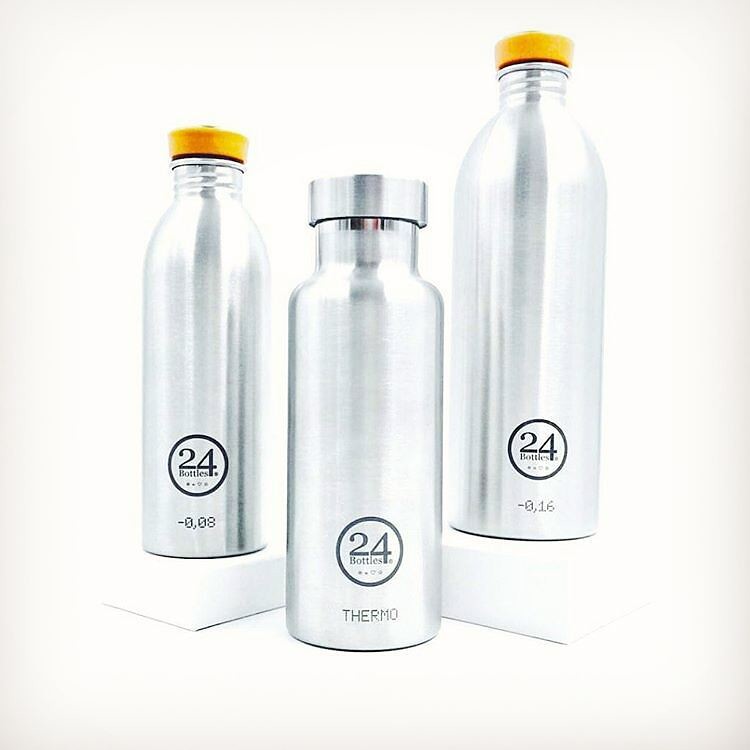The advertisement features a set of three stainless steel, reusable water bottles with a shiny, reflective silver finish, photographed against a pristine white background. The bottles are positioned on three different levels, reminiscent of a winners' podium, imparting a sporty and competitive feel to the arrangement. The bottle in the center, which has a wider body and square shoulders, is adorned with the "Thermo" logo and a "24" marking. It also sports a larger, flatter silver mouthpiece that screws on. The bottle on the left is smaller, perched on a white stand, and marked with "-0.08" and the "24 bottles" logo within a circular emblem. It features a rounded shoulder and a mustard-colored twist-on cap. Similarly, the bottle on the right is also elevated on a white base, marked with "-0.16" and the same "24 bottles" circular logo, featuring rounded shoulders and a mustard-colored twist-on cap. All three bottles glisten under the light, emphasizing their high-quality metallic finish and modern design.